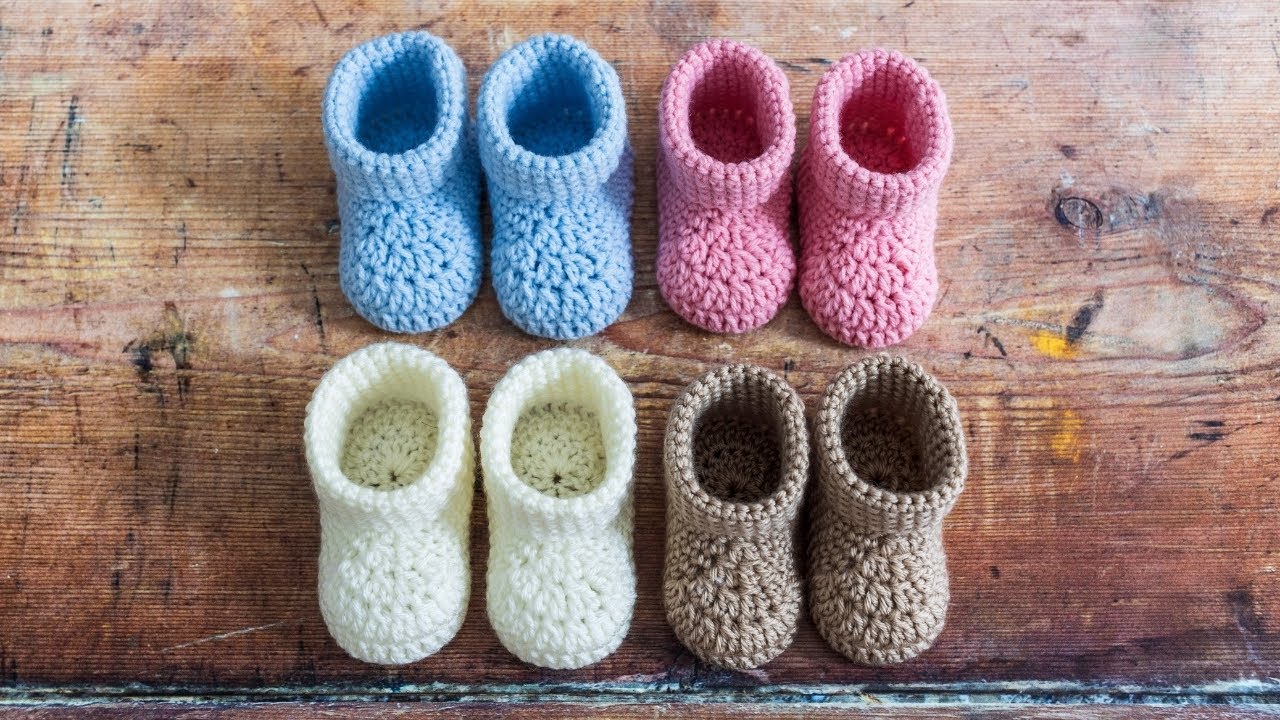This indoor photograph, captured in a photographic style from a bird's-eye view, focuses on four pairs of knitted baby booties. The booties, arranged in two neat rows on a light wood table or bench with noticeable wear and markings, showcase a soft and cozy texture. From left to right, the top row features a pair of light blue booties followed by light pink ones, while the bottom row includes white booties adjacent to light brown booties. The booties, characterized by their crocheted design with small cuffs at the openings, appear set on a worn surface marred with black pen-like marks to the left and yellow stains to the right, complemented by a grey streak running along the bottom. The overall scene presents a charming yet rustic tableau of baby footwear against a slightly weathered wooden backdrop.